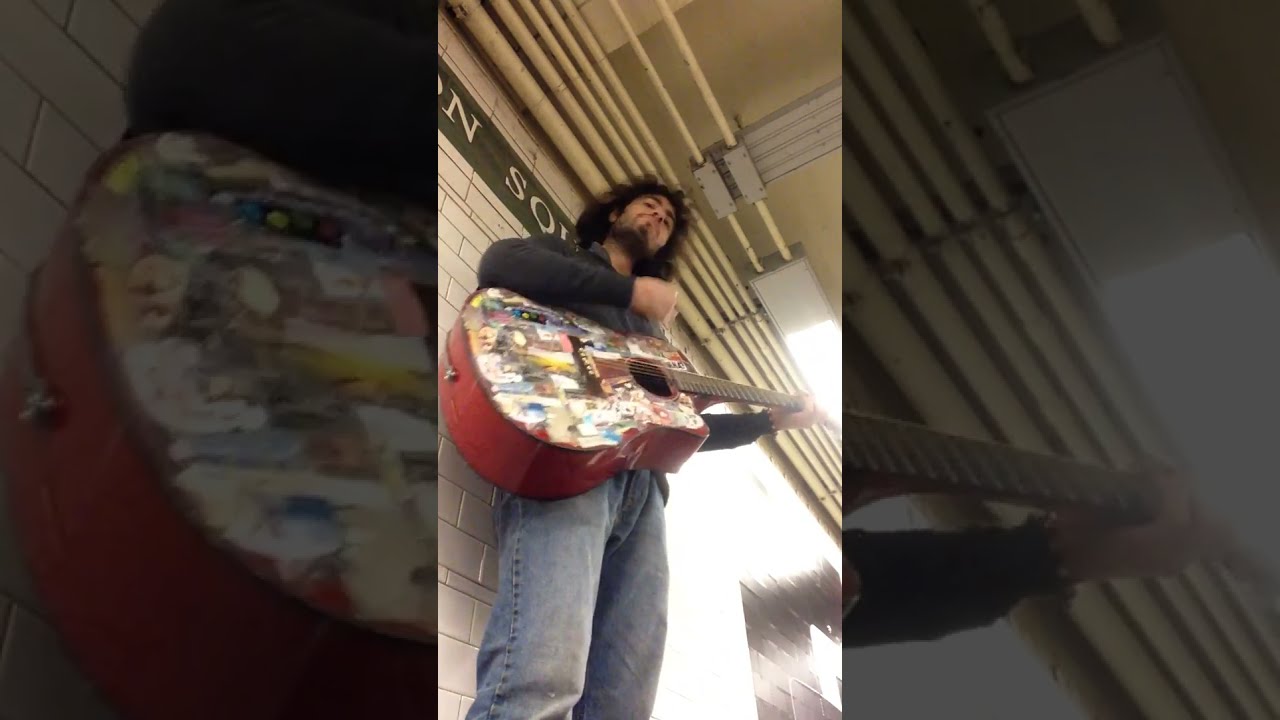The image captures a unique upward perspective of a man playing a wooden acoustic guitar, heavily decorated with a collage of stickers on its face. The photograph, taken inside a building, features the man standing above the viewer, who might be sitting on the floor. He has fair skin, thick, poofy dark curly hair that reaches his shoulders, and a black beard visible from beneath his chin. He is dressed in a long-sleeved black shirt and loose-fitting light blue jeans. Behind him is a wall lined with white tiles in a brick pattern, and a black banner with white lettering—partially reading "N S" and possibly "C" or "O"—angles down in the upper left corner. The ceiling is intersected by multiple pipes and some gray casing. The overall setting gives off a vibe reminiscent of a train or subway station, suggesting he might be busking in such a location.